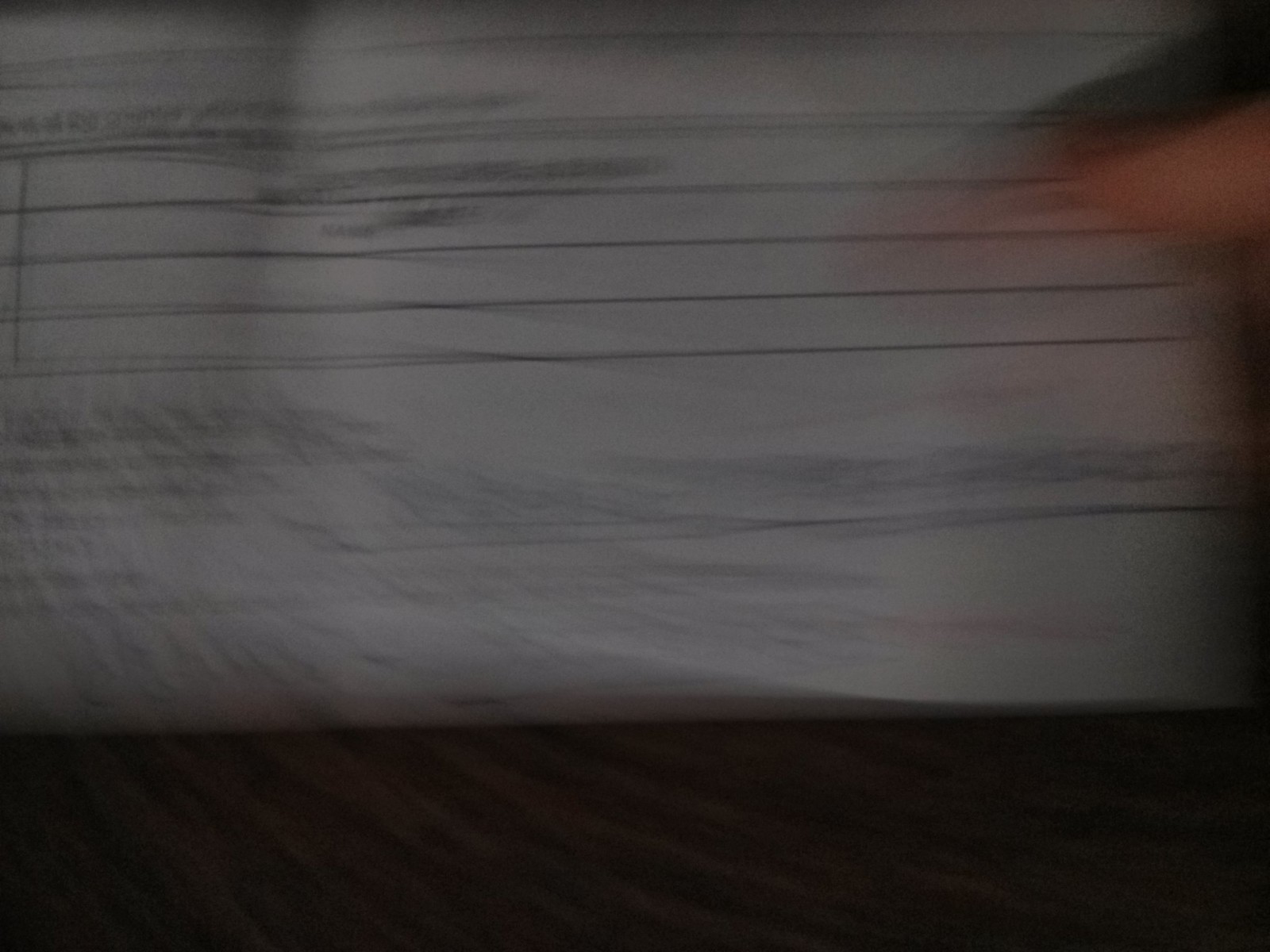The image captures a blurry scene, likely taken with a camera or cell phone in motion. The primary subject appears to be a person filling out a form on a desk made of dark wood. The wood grain is visible in the lower part of the image. On top of the desk lies a white sheet of paper covered in black text, suggesting that it is a printed form. In the upper right corner, a hand—potentially with a thumb and forefinger grasping a dark-colored pen—is visible, indicating active writing. The form showcases numerous lines and handwritten information, primarily concentrated on the left side of the image. Overall, the photo has a darker, somewhat shadowed appearance, adding to its unclear quality.